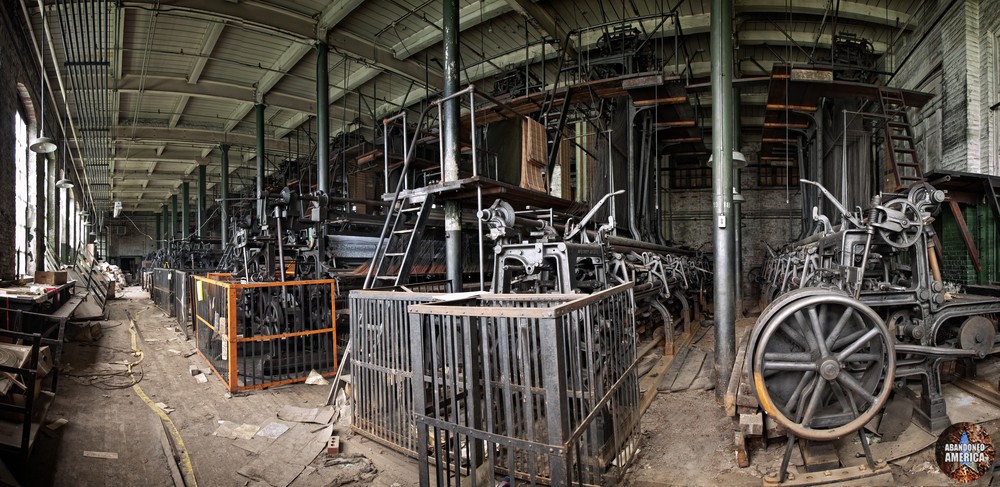This color photograph, taken indoors during the daytime, depicts an abandoned, early 1900s-era factory. The factory interior is dominated by long rows of old industrial machinery, including wheels and belts, stretching from right to left. The foreground reveals a dirty, reddish-rust colored floor littered with scattered papers. The background features brick walls and white ceilings with a grid-like pattern formed by rims and ridges, supported by steel pillars and columns. A ladder leans against one of the pillars, while metal steps lead to a second floor. Near the center-left of the image, there's a collection of metal cages, one with a wooden trim. The image, marked with a small "Abandoned America" logo at the bottom, evokes the sense of a once-bustling manufacturing plant, possibly a printing press room, now eerily silent and unused for years.